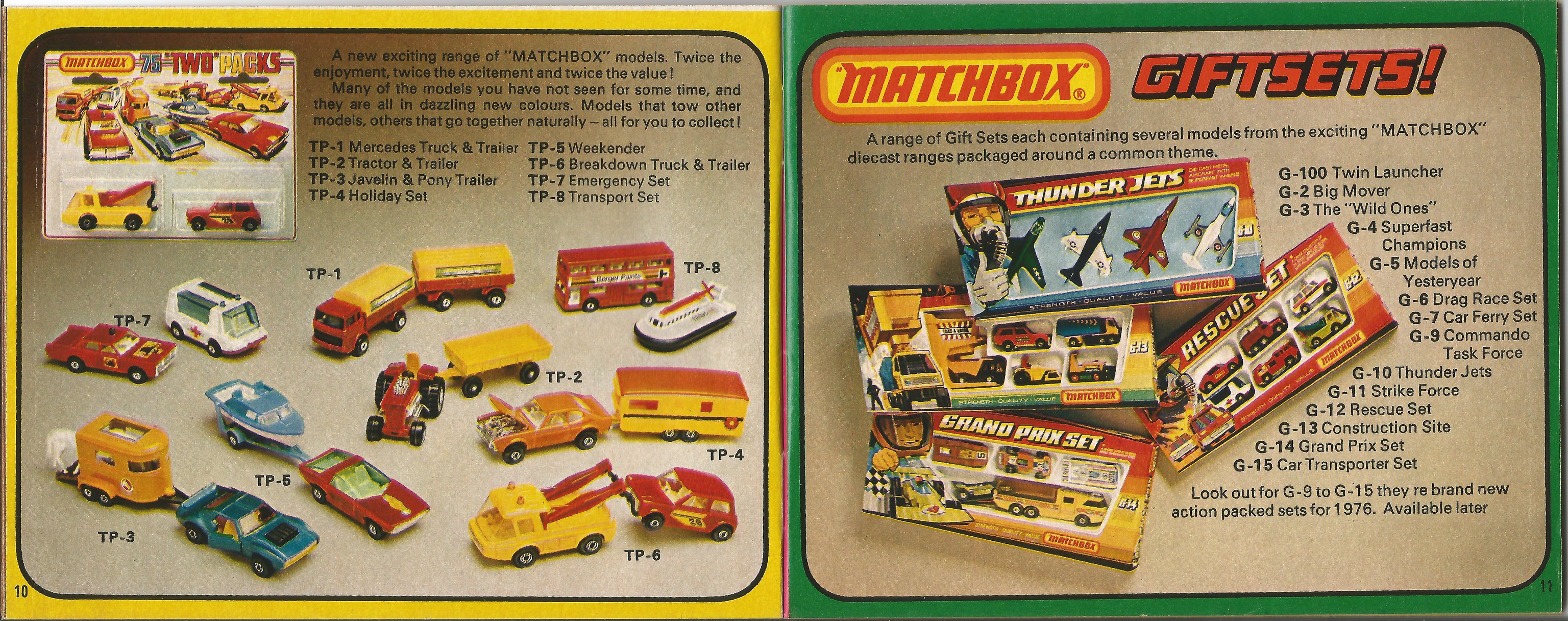This image appears to be a two-page advertisement for Matchbox toy cars, presented as an open pamphlet. The left page is outlined in yellow and displays a variety of Matchbox cars in different colors, along with small-font descriptions. The right page, bordered in green, prominently features the heading "Matchbox Gift Sets" at the top, followed by descriptions and small wording detailing four distinct gift sets: Thunder Jets, Rescue Set, Trucks, and Grand Prix Set. The gift sets are illustrated with rectangular boxes showcasing colorful miniature vehicles, including planes, trucks, a red bus, a car towing a trailer, and an ambulance. The vibrant toy cars are depicted in colors such as red, orange, yellow, blue, and white, capturing the playful and diverse range of Matchbox products advertised.